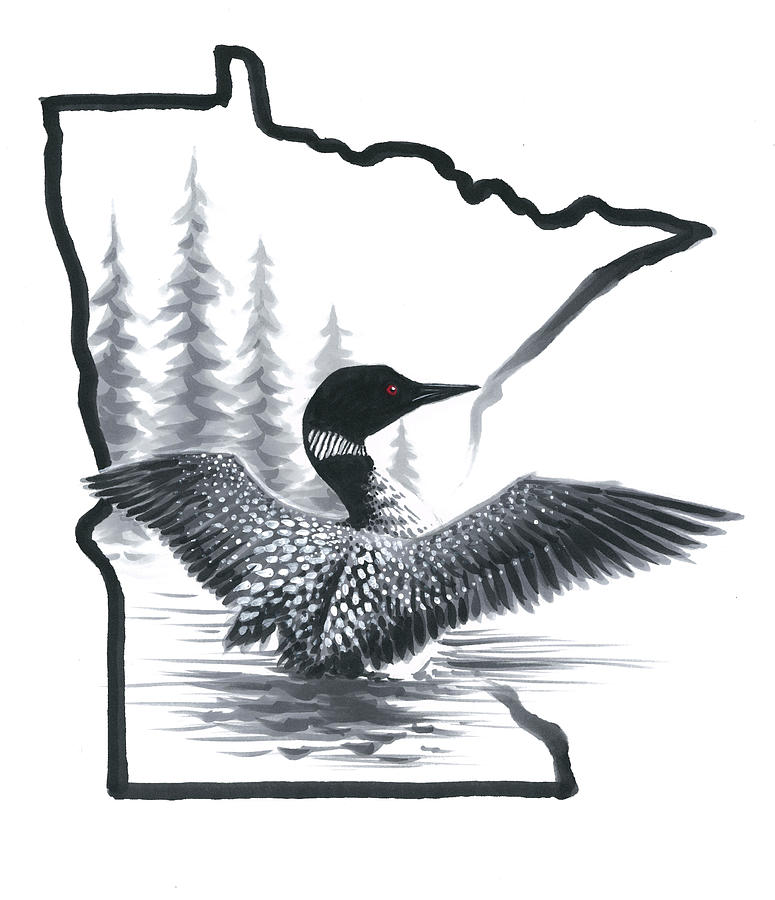This black and white hand-drawn image depicts a bird, likely a duck or the state bird of Minnesota, partially submerged in water with its legs underwater and its body and spread wings above. The bird is viewed from behind, showcasing its mostly black and gray wings adorned with white spots. It has a striking red eye, the only colored element in the drawing. The bird's neck features diagonal white stripes against a black backdrop, and its black head contrasts sharply with its red eye. Surrounding the bird is an outline of the state of Minnesota, incorporating the silhouettes of large pine trees. The water body the bird floats in merges seamlessly with the white background of the image. The entire drawing is bordered by a uniquely shaped outline resembling a jigsaw puzzle, adding an intriguing frame to the serene nature scene.